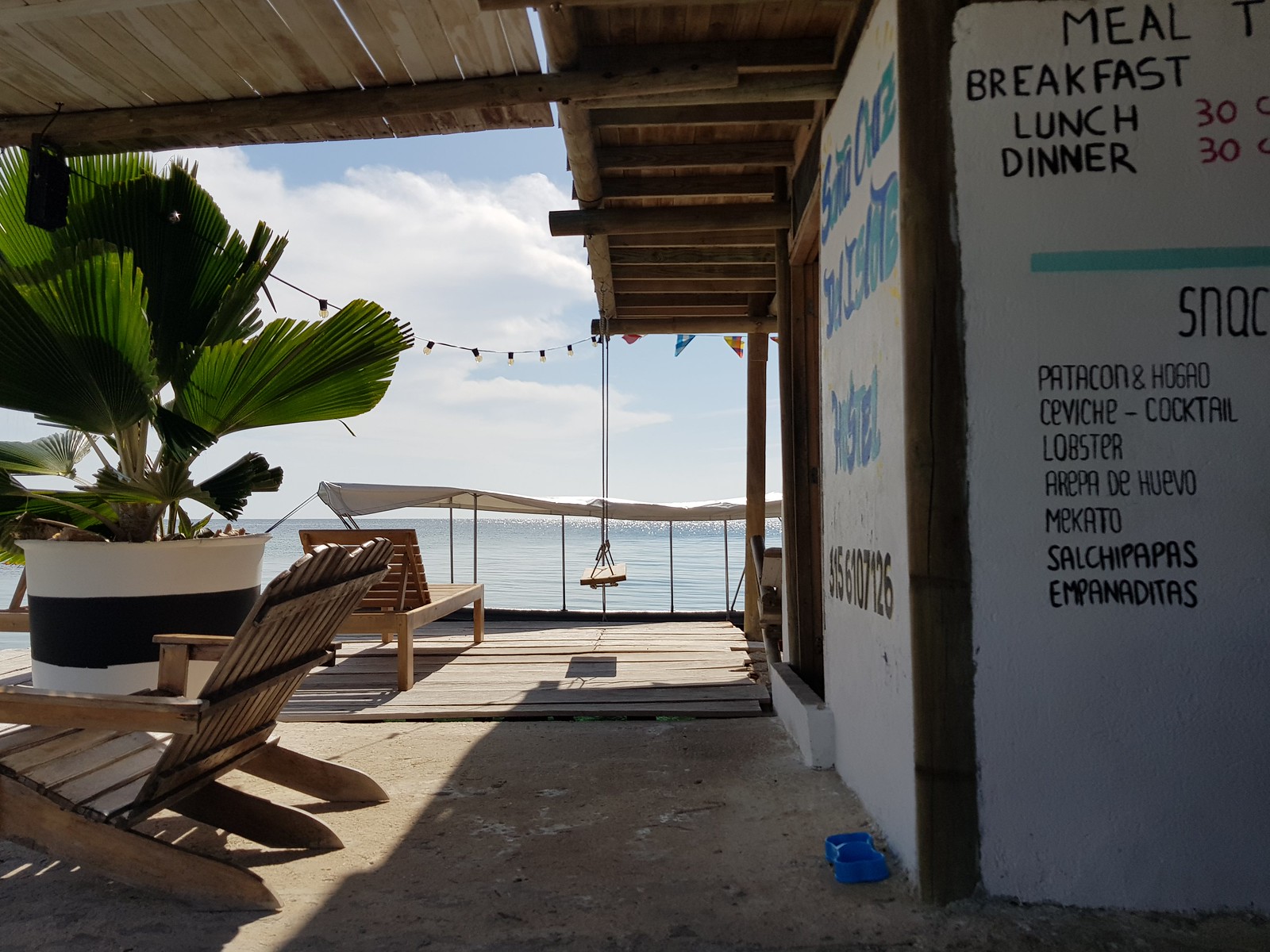The image showcases a quaint little food shack situated on a beachfront, possibly a charming restaurant with a tropical ambiance. The covered patio of the restaurant extends out towards a pier overlooking a clear, blue body of water, accentuated by a light blue sky scattered with puffy clouds, hinting at a serene summer or spring day. 

On the right-hand corner of the white building adorned with blue trim, there is a dark brown menu board displaying meal options for breakfast, lunch, and dinner, along with various snacks. The text is slightly obscured due to the angle, but some menu items like cocktails, lobster, macato, and empanaditas, suggest a diverse, potentially Mexican, cuisine. 

In the forefront, a cozy seating area features both wooden beach chairs on a combination of concrete floor and wooden deck. A lush green palm plant in a striking white planter with a black stripe adds to the tropical feel. Large white umbrellas dot the patio, providing shade and enhancing the inviting atmosphere of this beachfront retreat.